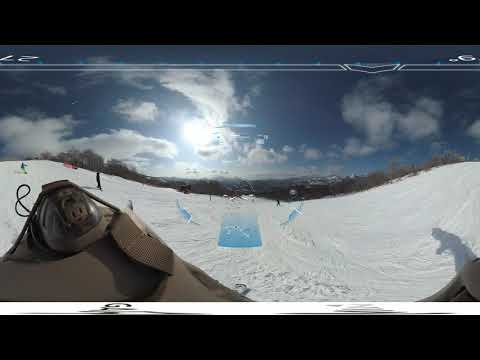The image captures a dynamic scene at a ski resort from the point of view of a skier, potentially with a GoPro. In the lower half of the frame, a brown bag, possibly a brown helmet, and some indistinct equipment are visible, along with the shadow of the person taking the picture, who appears to be holding ski poles. There are snowy hills populated by both skiers and snowboarders, primarily on the left side and center of the image. The ski slope is bustling with activity as people descend the hill. In the background, the vast, snowy mountains stretch into the distance under a partly cloudy, yet brilliantly illuminated blue sky. The sun, slightly left of center, bathes the entire scene in bright light. At the top of the image, numbers 27 and 9 appear upside down on either side, likely part of the camera's interface or display. The overall composition showcases both the serene beauty of the snowy landscape and the lively atmosphere of the ski resort.